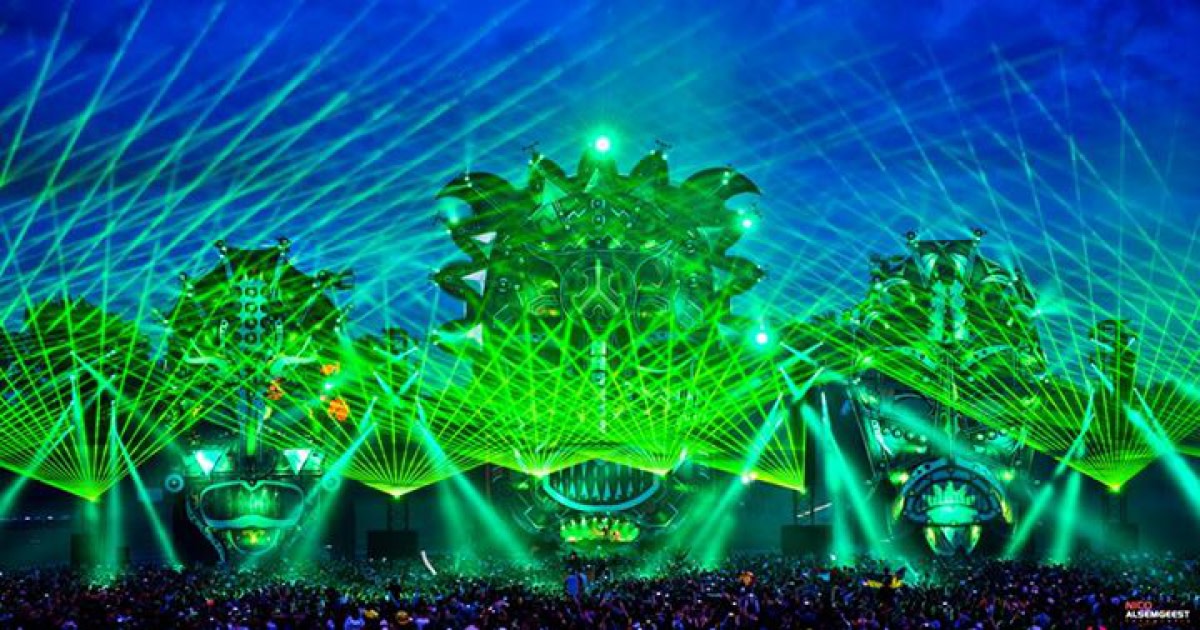The image captures an outdoor concert scene with dazzling green laser light effects and a massive crowd packed shoulder to shoulder. Five adjacent stages, each adorned with intricate metal beams, dominate the scene. Green lights emanate from these beams, creating a spectacular display of geometric shapes and grids against a cobalt blue sky dotted with clouds, perhaps an hour after sunset. The illuminated frames above each stage shoot greenish, whitish lasers skyward, intersecting to form mesmerizing patterns. Floodlights also cast a green glow over the crowd, enveloping them in the vibrant spectacle. Amidst the stunning light show, the intricate temple-like structures atop each stage add to the grandiosity, making the scene appear almost computer-generated in its surreal brilliance.